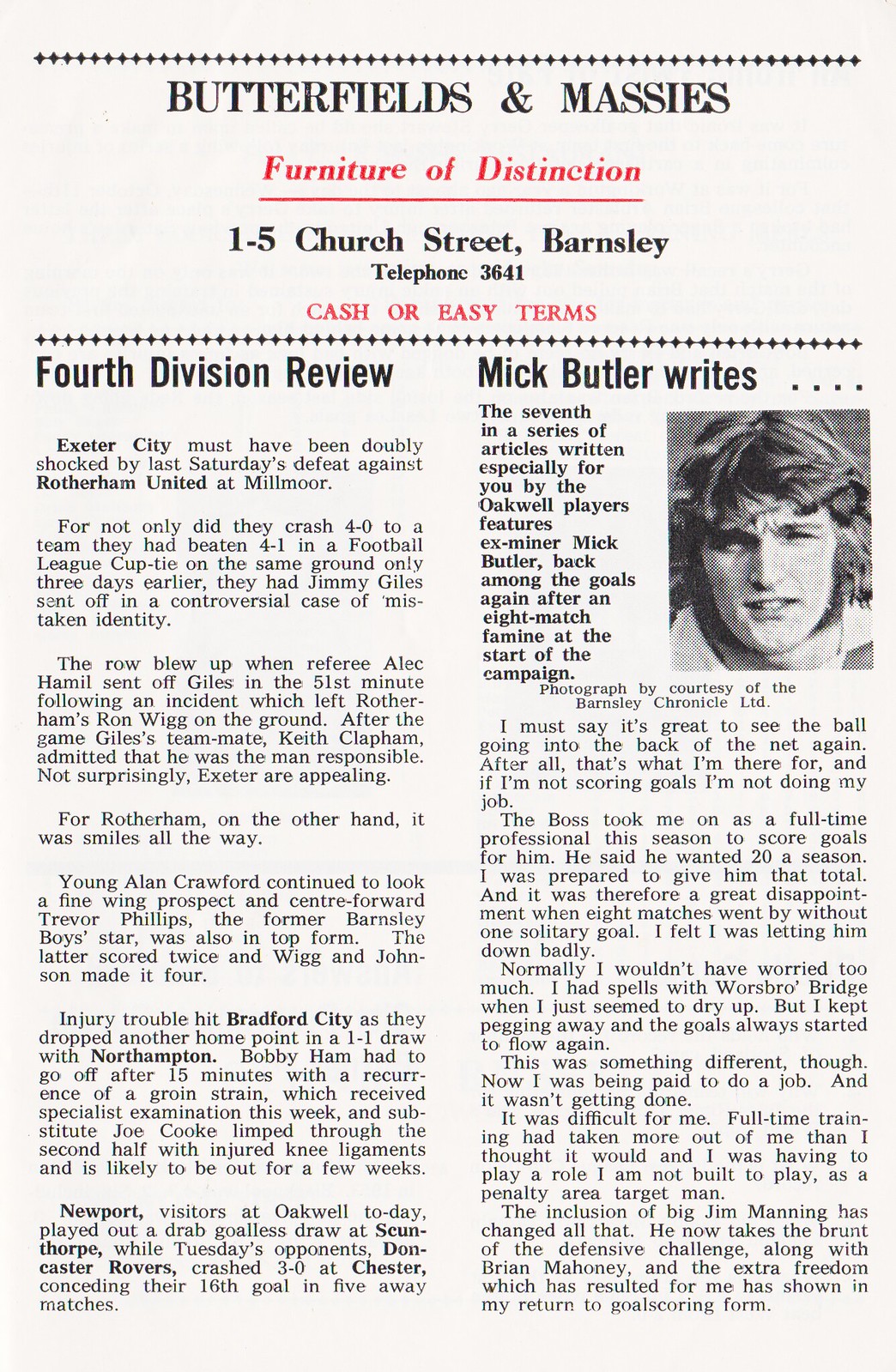The image is a detailed scan of an entire newspaper page, predominantly black with tan, red, white, and different shades of grey. The page is divided into two columns of text with a black-and-white photo of a man with medium hair and a white complexion situated on the middle right side. At the top of the page, there's a bold banner titled "Butterfields and Massey's" in a serif black font, followed by "Furniture of Distinction" in underlined red italics. Below this, the address "1-5 Church Street, Barnsley, Telephone 3641," is printed in black, with "Cash or Easy Terms" in red all-caps directly underneath. The left column features a sports article titled "4th Division Review," detailing Exeter City's shocking 4-0 defeat against Rotherham United, a team they had previously beaten 4-1 just three days earlier in a Football League Cup tie on the same ground. The article discusses the controversial sending off of Jimmy Giles due to a case of mistaken identity. Further down, the heading "McButler Writes..." indicates another section of commentary. The page is consistent with the design and content of a vintage sports newspaper.